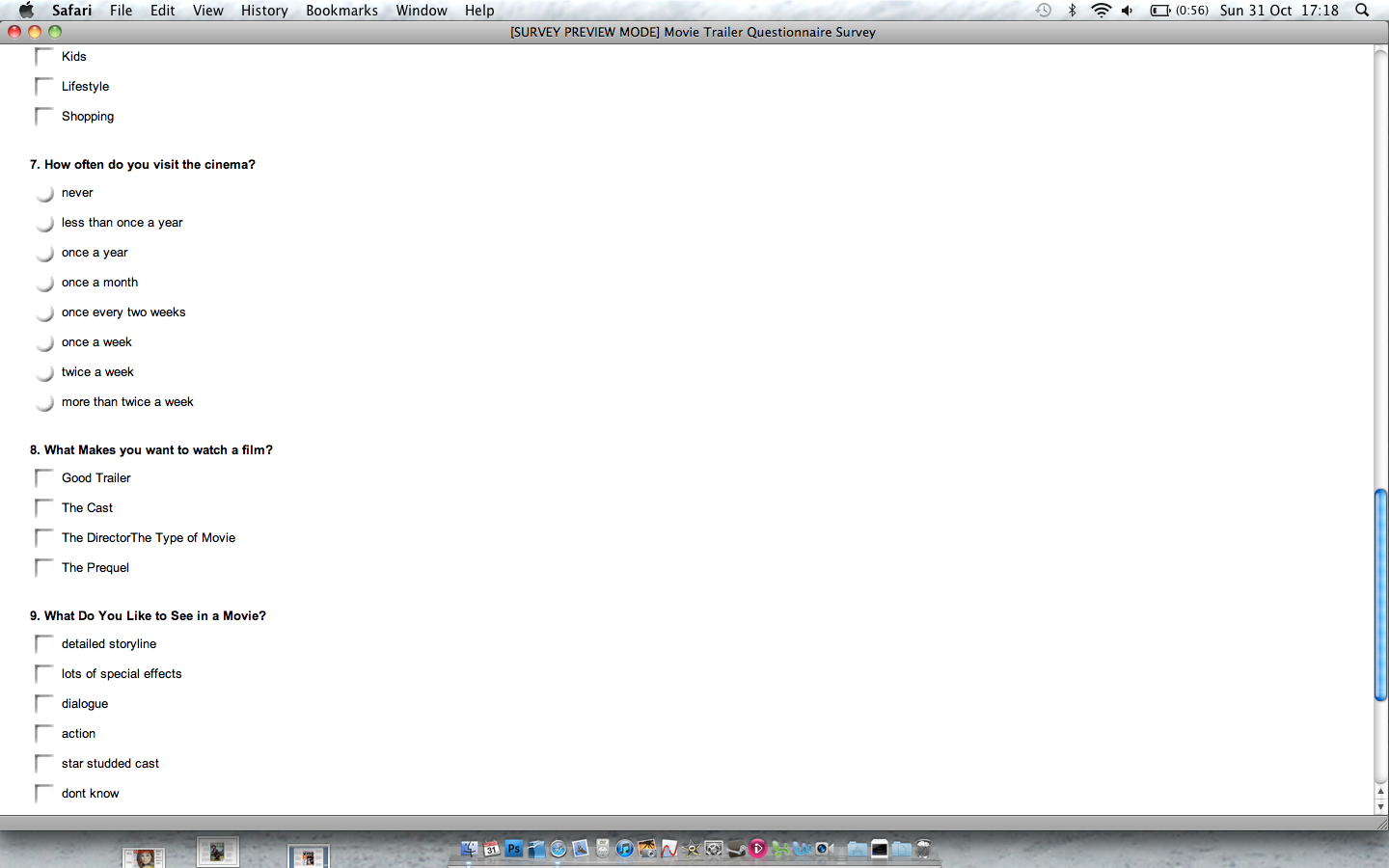This is a detailed screenshot taken from the Safari browser on a macOS interface. The image features a thin, cloud-gray border. At the very top, the familiar Apple icon is displayed, followed by black text listing the Safari menu options from left to right: Safari, File, Edit, View, History, Bookmarks, Window, and Help. 

On the upper-right corner, standard macOS icons are neatly lined up, including a search icon, the current time and date, battery percentage indicator, sound toggle, Wi-Fi status, and Bluetooth connection icon.

Just below this is a slightly darker gray border, visible on the left side, featuring typical window control buttons: a red circle (close), a yellow circle (minimize), and a green circle (maximize). In the center of this border, in black text and parentheses, it reads "Survey Preview Mode." Below, the text titles the survey as "Movie Trailer Questionnaire Survey."

Underneath the window control buttons, there are several black-bordered white squares aligned vertically with accompanying labels: "Kids," "Lifestyle," and "Shopping."

Featured prominently in bold black text is question number seven: "How often do you visit the cinema?" Under this question, a series of small circles form a vertical list, each circle indicating a multiple-choice answer. The options listed are: 
1. Never
2. Less than once a year
3. Once a year
4. Once a month
5. Once every two weeks
6. Once a week
7. Twice a week
8. More than twice a week

Below question seven, number eight asks, "What makes you want to watch a good film?" followed by four selectable answers. Question nine reads, "What would you like to see in a movie?" with six additional choices available for selection.

At the bottom of the screenshot, a gray border spans across, containing numerous small icons, though their details are indistinct and difficult to discern.